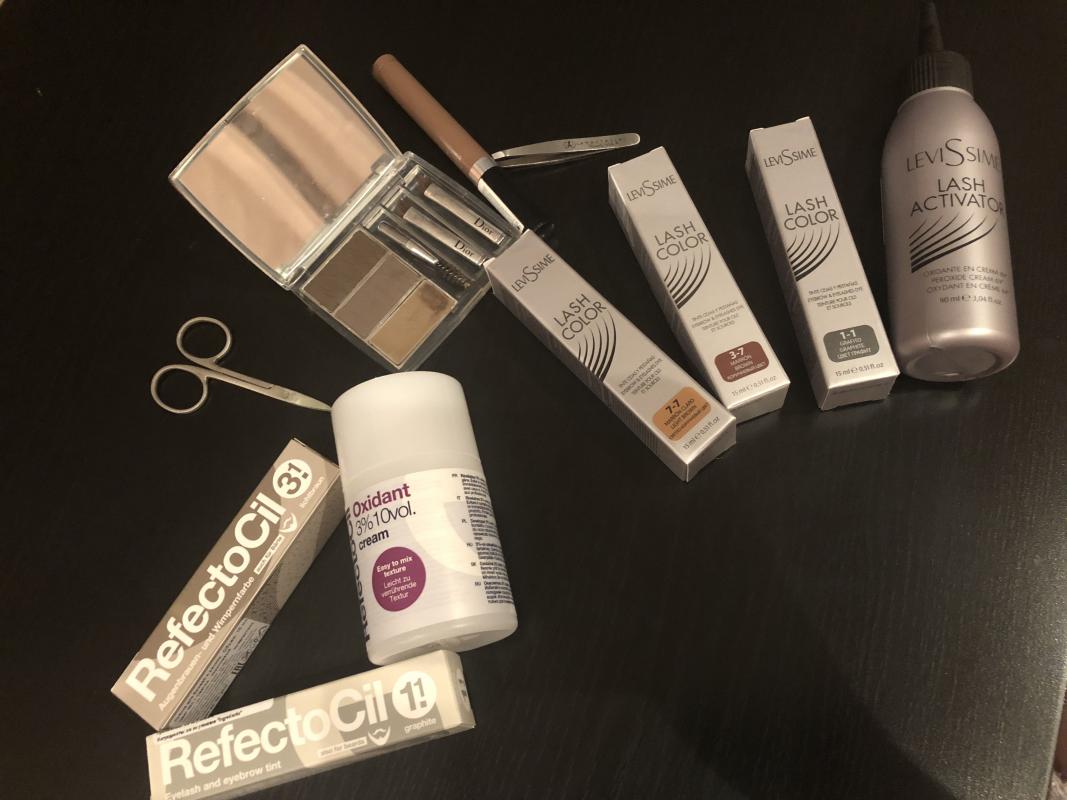The image showcases a curated selection of nine makeup products meticulously arranged against a sleek black background. Starting from the upper right-hand corner, the display features a silver bottle labeled "Lash Activator." To its left, there are three slim white rectangular boxes labeled "Lash Color," organized sequentially with each featuring an image of an eyelash and color codes at the bottom indicating the shade of the product.

Adjacent to these boxes is an open eyeshadow palette. The palette's top cover has a mirror, and within the palette, there are three eyelash colors on the left side and three stick colors on the right side. Positioned next to the palette is a small pair of scissors, suggesting the precision required for makeup application.

Additionally, there is a jar prominently labeled "Oxidant 36%, 10 VOL cream." Leaning against this jar, you find two tube containers inscribed with "RefectoCil 3.1" and "RefectoCil 11," respectively. The placement of these items not only highlights their use in eye makeup but also their complementary nature within a professional makeup routine. All products are encased in stylish silver and white containers, reinforcing a sense of elegance and sophistication.